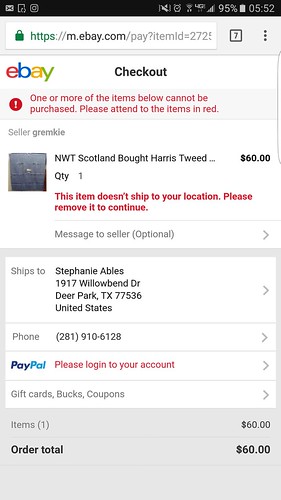The image is a rectangular snapshot taken from a cell phone, oriented vertically. At the top, there is a black status bar containing several white icons: a Gmail notification, two unidentifiable icons on the left, a muted sound icon, an alarm icon, another unrecognized symbol, a "4G" label, a cellular signal indicator showing 3 out of 4 bars, a 95% full battery icon, and the current time displayed as 05:52. Below this, there is a gray banner featuring a URL box with "m.ebay.com". Next to the URL, there is a white box with a black outline displaying the number 7, followed by three vertical dots.

The subsequent section displays the eBay logo and the word "Checkout". Below this, a red warning message with an exclamation point indicates that "one or more of the items below cannot be purchased. Please attend to the items in red." The seller's username "Grimkli" is listed afterward, accompanied by a small image, though the contents of the image are indistinguishable. The item detailed is "NWT Scotland bought Harris Tweed," with a quantity of one and a price tag of $60. The warning in red below states, "This item doesn't ship to your location. Please remove it to continue."